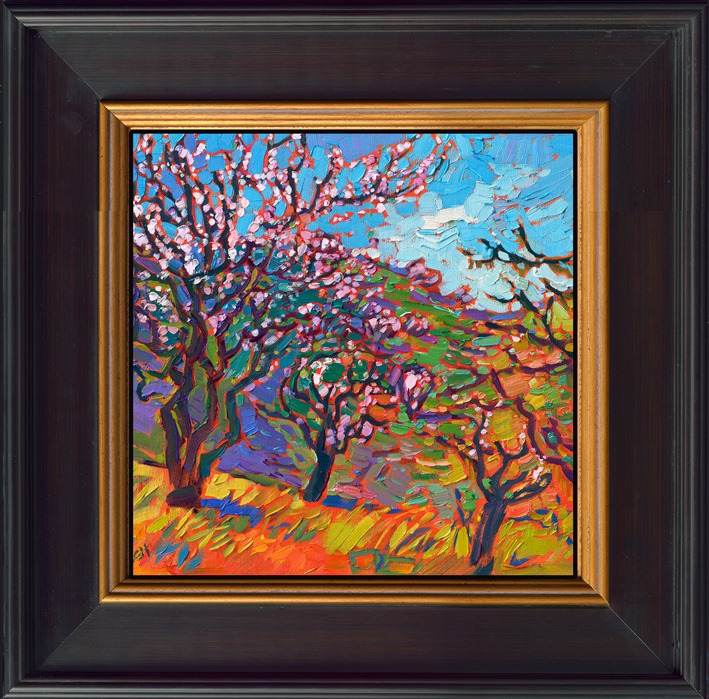A vibrant framed painting is depicted in this image. The frame is a dark, almost black, deep brown wood with a thick, crown molding design, encasing an inner golden trim. The painting itself is a colorful abstract representation of nature. It features multiple trees with a variety of colors. On the left side, a close-up tree displays white, orange, and purple leaves with a grayish-black trunk flecked with green. In the middle background, another tree with a dark blue-black trunk and spots of purple and green stands. To the right foreground, a smaller tree with sparse white leaves is visible. The ground is painted with yellow, blue, orange, and green hues, depicting a grassy field. Rolling colorful hills of green and purple stretch into the background, while the sky above is light blue with scattered white clouds, all rendered with thick, textured brushstrokes adding depth and dimension to the scene.